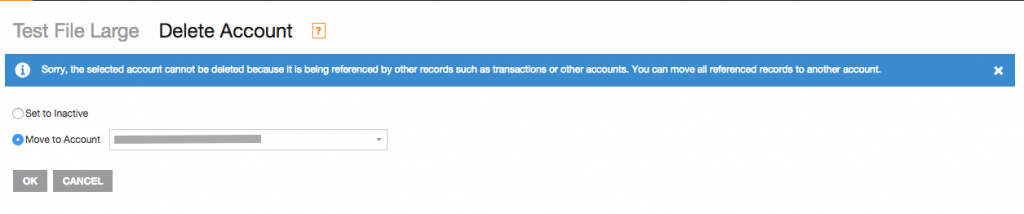The image displays a web page with a predominantly white background and minimal elements. At the very top, there is a thin black line stretching across the screen; a small segment on the top-left corner of this line is colored orange. Below this, in larger gray font, are the words "Test File Large". To the right, in black text, are the words "Delete Account", and adjacent to these words is a small orange box containing a question mark.

Directly beneath this section is a blue horizontal bar that spans the entire width of the screen. On the right end of this bar, there's a white "X", and on the left, a white circle with a blue "i" inside it. The text within the blue band, written in white, states: "Sorry, the selected account cannot be deleted because it is referenced by other records such as transactions or other accounts. You can move all referenced records to another account."

Further down the page, returning to the white background, there are two choice buttons for selection. The first button, labeled "Set to Inactive", is represented by an open circle. The second button, labeled "Move to Account", has a blue circle with a white dot in the center, indicating it has been selected. To the right of these buttons, there is a response box featuring a down caret, with a gray line inside suggesting that information has been redacted or is blank. Below these elements, on the left, is a gray button with the word "OK" in white text, and to the right, another gray button with the word "Cancel" also in white text.